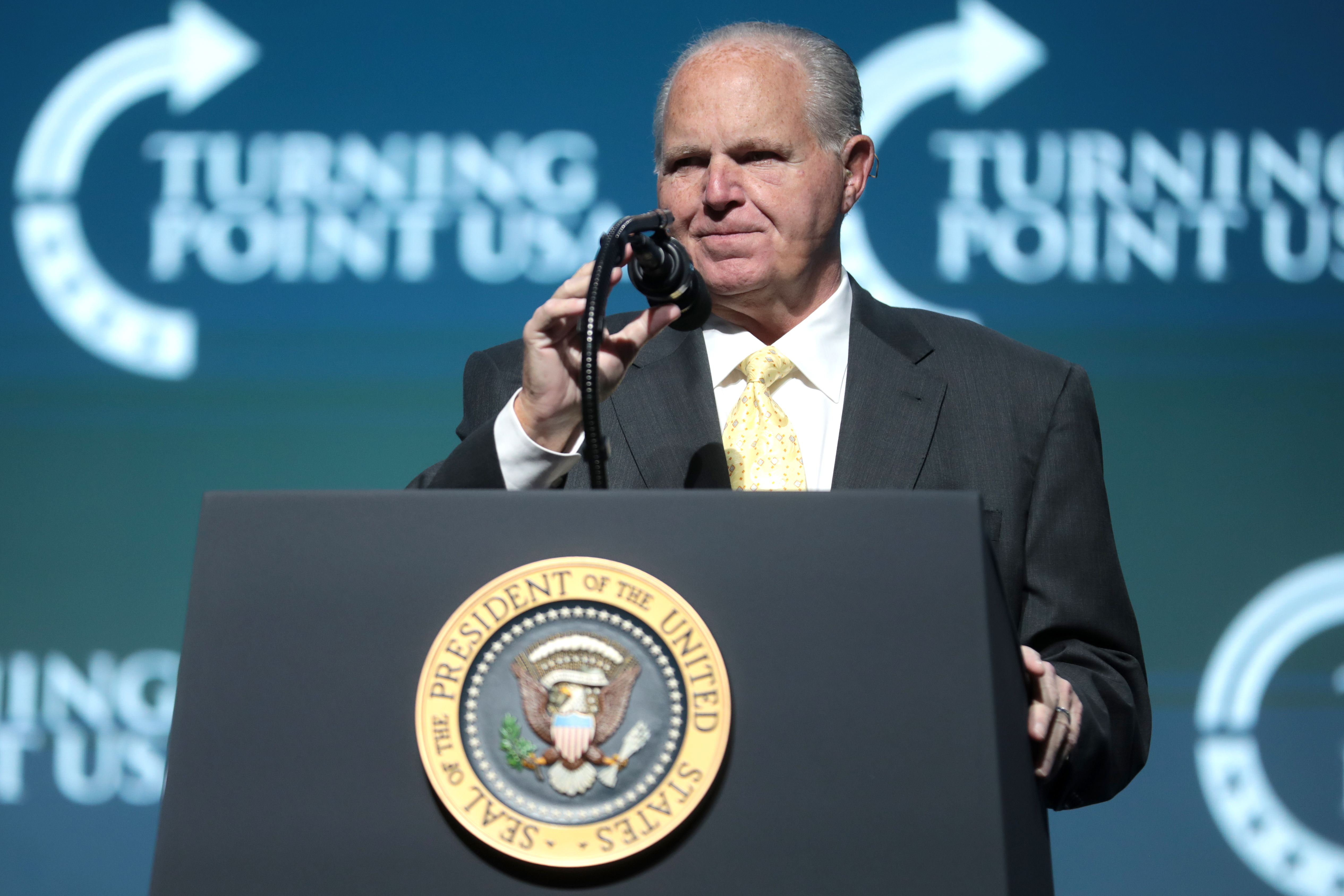In this detailed photograph, Rush Limbaugh stands behind a dark black-blue podium, prominently featuring the seal of the President of the United States in gold with black lettering. The seal showcases an American Eagle, clutching arrows and an olive branch in its talons. Limbaugh, appearing older with thinning, slicked-back gray hair, is dressed in a black suit, a white button-up shirt, and a yellow tie. Holding a black microphone with his right hand, he seems to be adjusting it, possibly bringing it closer to his mouth. His left hand is gripping the podium on the right side of the image. Behind him, the backdrop is a blue-green hue, adorned with the repeated logo of Turning Point USA, featuring white lettering and a circular, curvy arrow.